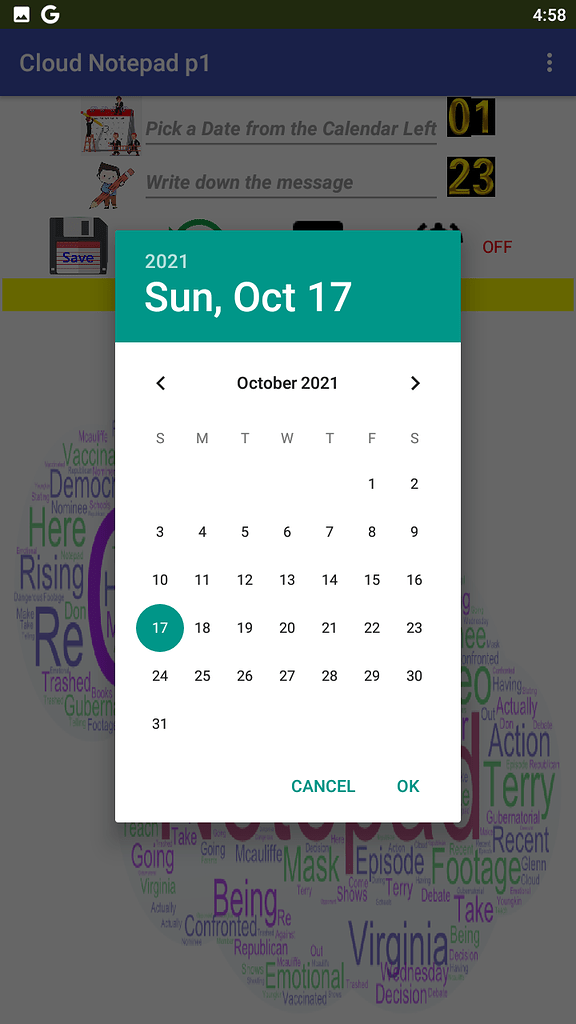## Descriptive Caption for the Screenshot

This screenshot, taken from an Android device at 4:58 PM on Sunday, October 17th, 2021, displays a detailed view of several elements on the screen. The primary focus is a calendar widget centered on the screen, with the date October 17th highlighted. The calendar features a green border at the top and green text at the bottom, possibly indicating additional information or options related to time zones.

Beneath the calendar, a word cloud is prominently displayed. The word cloud includes terms such as "Virginia" and "being," alongside various other words, though the source of these words is unclear. The word cloud is saved as a file titled "Cloud Notepad P1," and its interface includes three vertical dots suggesting the presence of additional menu options or further details.

In the upper section of the screenshot, various Google IDs and additional tabs are visible, indicating that the user may have multiple accounts or open applications. Overall, the image captures a moment in time where the user appears to be interacting with the calendar and the word cloud application, possibly to select a date and jot down relevant information.